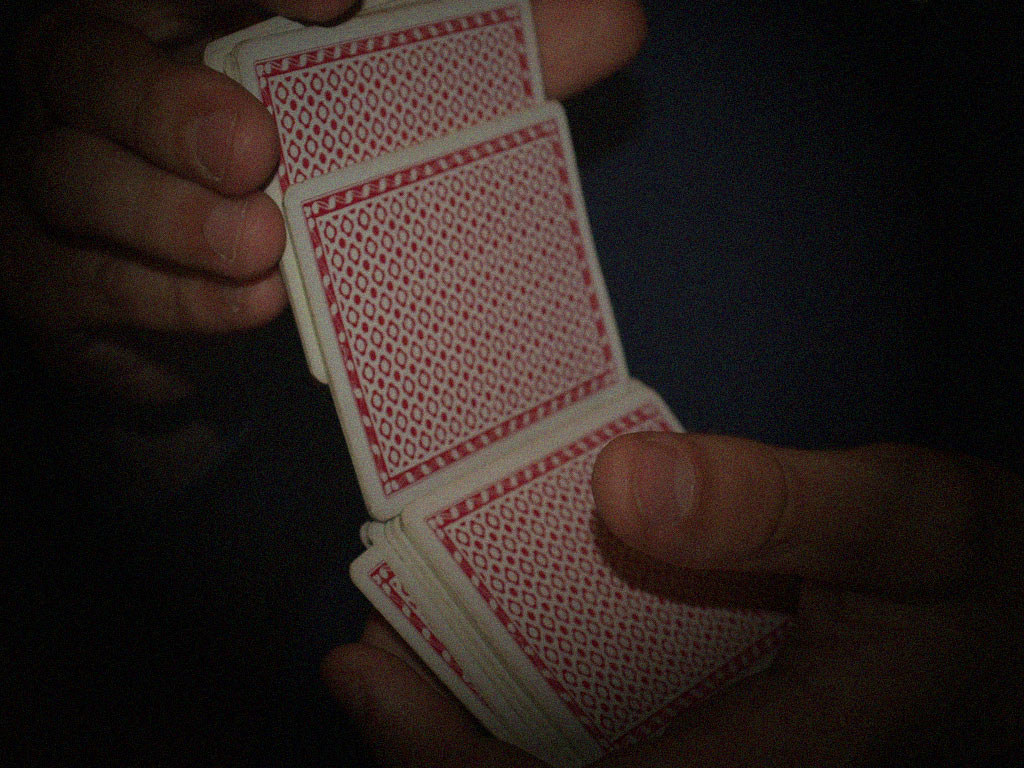The image features a close-up view of a man's hands against a black background, expertly shuffling a deck of cards. The cards are designed with a nostalgic touch, featuring a white background adorned with intricate red detailing. Each card showcases a large red border around the edges, filled with tiny white figures. The main design consists of a continuous pattern of red diamond shapes with small dots between them, creating a visually striking and classic appearance.

One of the man's thumbs firmly holds down the bottom of the deck while his fingers wrap around the side, securing the cards in place. Among the neatly aligned cards, one has slightly slipped out of order, adding a touch of dynamic realism to the scene. His other hand hovers above the deck, guiding the cards as they cascade from one hand to the other in a rhythmic shuffling motion. The image beautifully captures the careful precision and skill involved in the act of card shuffling.